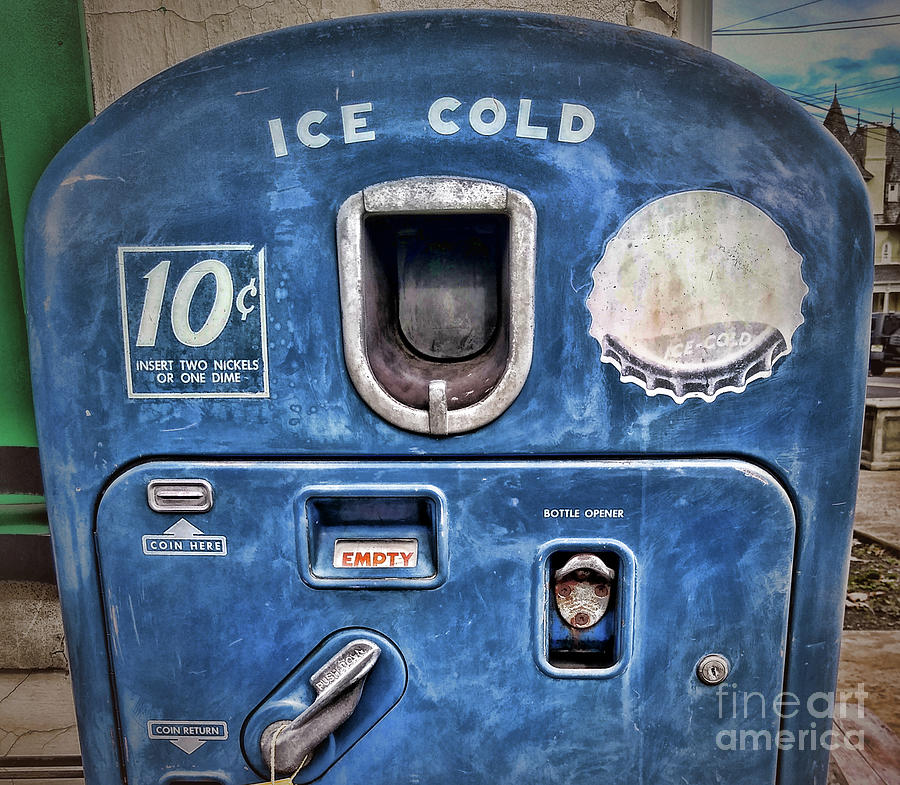This detailed artwork is a close-up depiction of a vintage ice machine. The main body of the machine is rectangular with a curved top, boldly labeled "ICE COLD" in capitalized white text. Central to the design is a small tray and hatch where the bottles of soda would emerge. On the right side of the machine, a faded bottle cap with the text "ICE COLD" can be seen. To the left, there is a white square indicating the price of "10 cents," with further instructions to "insert two nickels or one dime." Below this, a small locked hatch marked "insert here" is present, along with an empty box space and a bottle opener next to a coin return slot. 

Fading into the background, the artwork transitions from a green wall on the left to a white wall, ending with a white building with black-tipped towers and peaks on the right. The lower right corner of the image features semi-faded text reading "FINE ART AMERICA." The meticulous attention to detail could make one initially believe it's a real machine, capturing the essence of vintage soda dispensers, complete with areas for coin insertion and bottle opening.